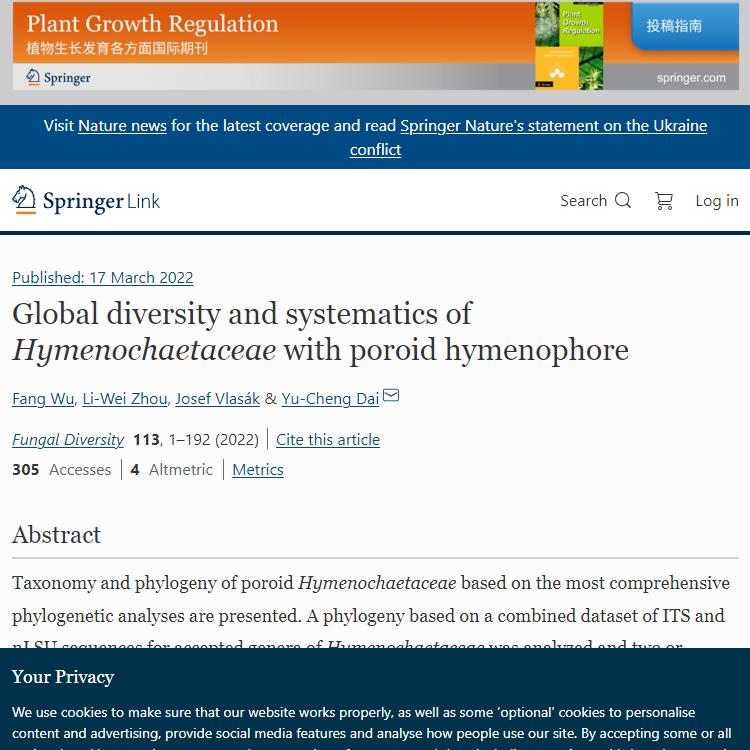Here is a refined and detailed descriptive caption for the image:

---

The image depicts a detailed screenshot of a website. At the top is a header with the text "Plant Growth Regulation" in white font set against an orange background. In the top right corner, there is a section of the header with a blue background and some text in an Asian language, which may include characters from Chinese, Japanese, or Korean writing systems.

Below the header, there is a banner with a blue background and white text that reads, "Visit Nature News for the latest coverage and read Springer Nature's statement on the Ukraine conflict." Immediately following, in blue text, is the link "Springer Link," positioned to the left of a search bar, a shopping cart icon, and a "Log In" option in gray font. A black line serves as a divider below this section.

Further down, there's the title of an article: "Published 17 March 2022: Global Diversity and Systematics of Hymenochatassia with Poroid Hymenophore" by four authors. Underneath the title, the publication details are in blue text, stating, "Fungal Diversity 113: 1-192 (2022). Cite this article," which indicates the article has had "305 accesses." To the right, there are links titled "Altmetric" and "Metrics."

Below this section is the abstract of the article, starting with a partial paragraph. At the very bottom, there's a footer that includes text about privacy, all set against a dark blue background with two sentences in white font.

---